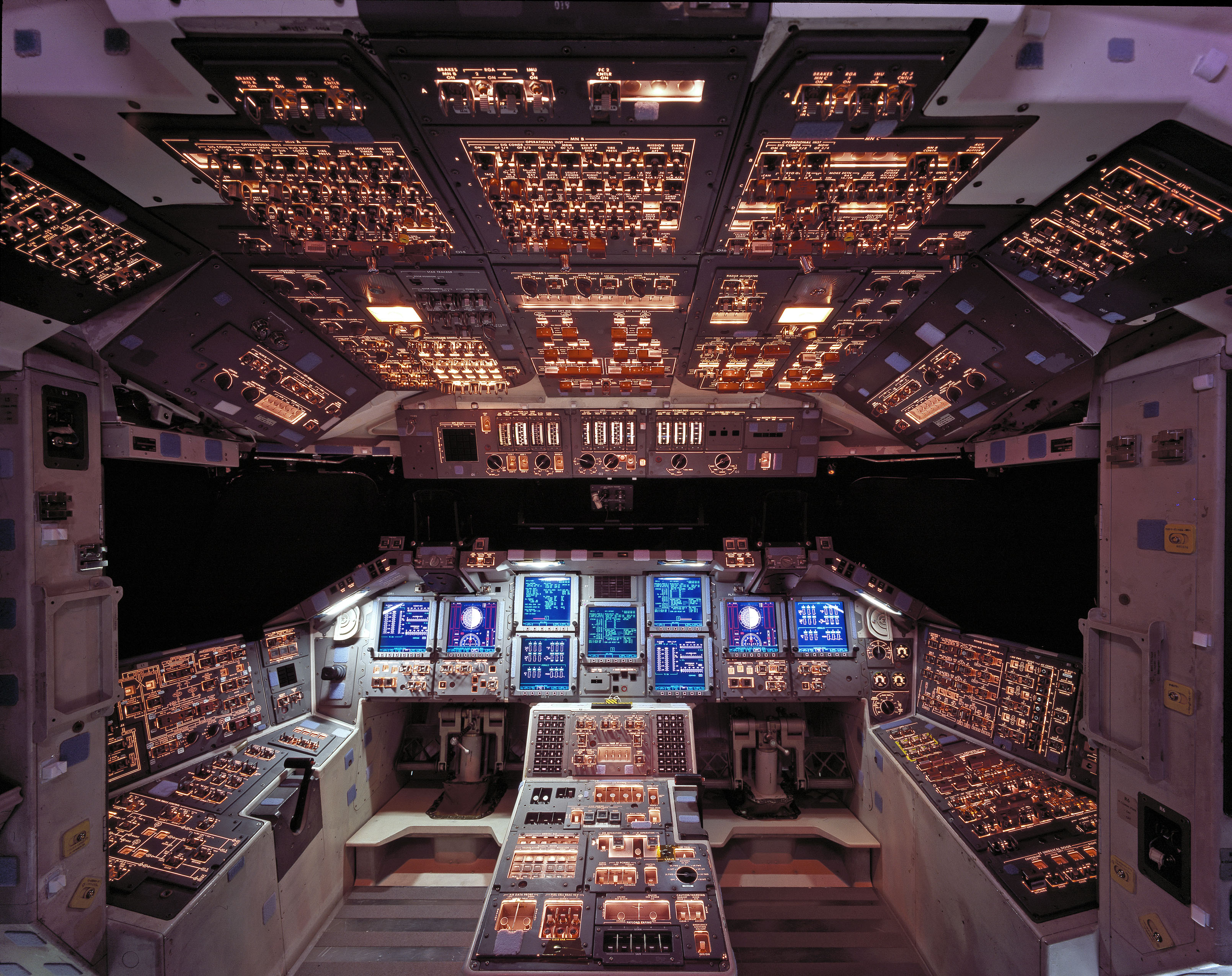The image depicts the intricate interior of a high-tech cockpit, brimming with controls and switches. The vantage point is from the rear, offering a sweeping view of the control panels at the front. The predominant colors are silver and black, with various sections illuminated, creating a striking visual contrast. A large, dark windshield dominates the front, though it offers no clear view beyond it.

Positioned below the windshield are numerous consoles fitted with blue screens displaying white readouts. These consoles are coupled with an array of illuminated amber switches and dials, distributed not just on the front panel but extending to the ceiling, sides, and central console. Surprisingly, there are no seats flanking the middle console, though the setup suggests there should be. Instead, situated beneath the central console is a complex mechanism, hinting at its potential operational significance with numerous mechanical dials and flip switches. This scene vividly resembles an aircraft cockpit, though the sheer volume of controls and readouts suggests it might belong to something far more sophisticated than a conventional aircraft.